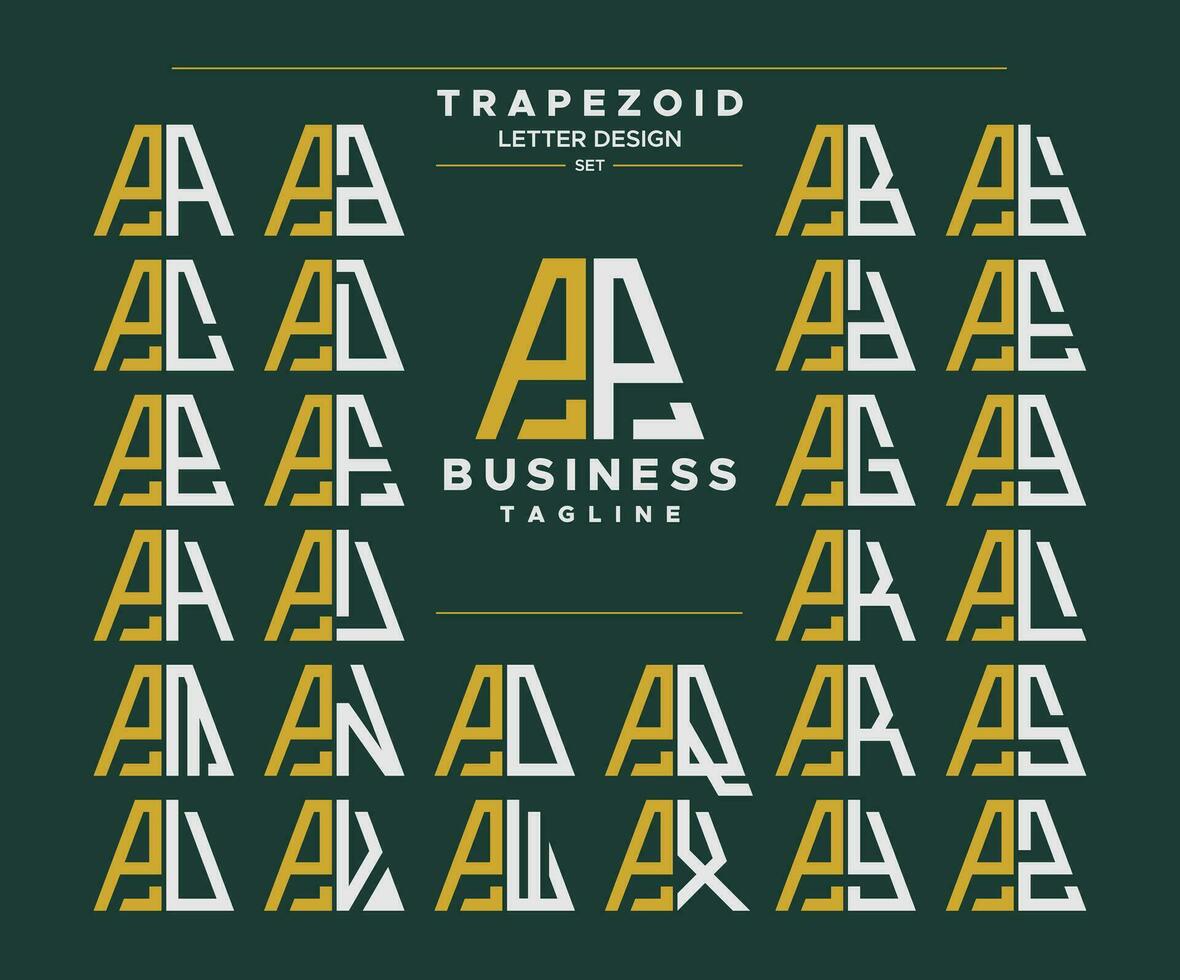This image features a square-shaped business card with a dark green, almost black, background. At the top, a thin yellow line stretches across, positioned about a centimeter below the edge. Below this line, bold white capital letters read "TRAPEZOID," followed by "LETTER DESIGN" and "SET" in progressively smaller fonts. The word "SET" is flanked by short greenish-yellow lines on each side. 

Centrally located is a logo comprising two interlocking letters, an "A" in yellow and a "white A", where the bottom corner of the "A" is detached and extends horizontally. Underneath this logo are the words "BUSINESS TAGLINE" in white uppercase letters. 

Below this, a smaller yellow line is positioned about an inch further down. Surrounding the central logo, on the left, right, and beneath, is a pattern featuring smaller iterations of the logo. These smaller logos form columns, with variations on the right side where the second letters change to different ones, creating combinations like A-C, A-D, etc. This pattern wraps around the central area almost entirely, except for the top portion. The overall design is complex and visually engaging, incorporating elements of repetition and symmetry to create a cohesive branding image.